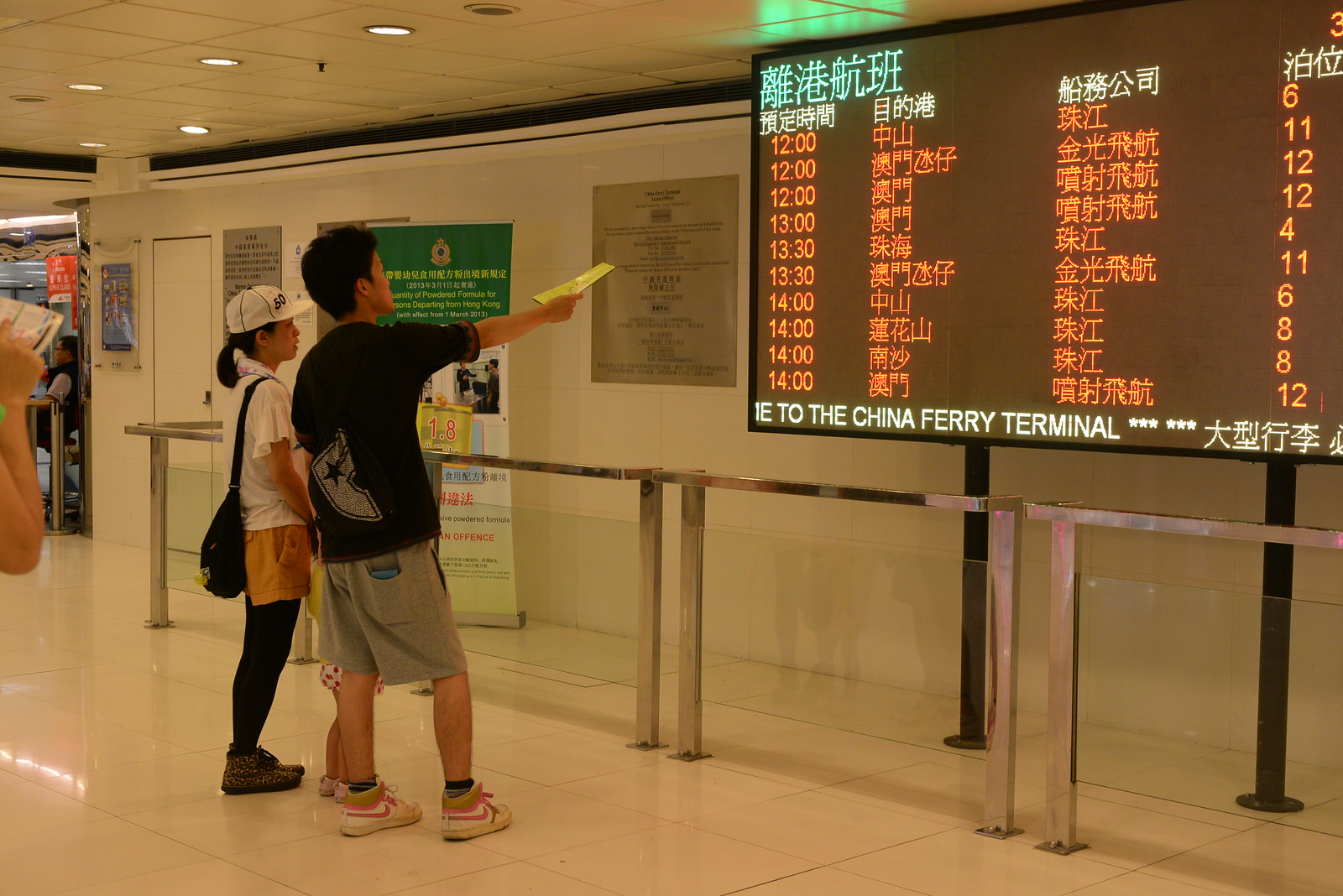In the image, we see a man and a woman standing at what appears to be a ferry terminal, indicated by the screen that reads "To the China Ferry Terminal." The duo, an Asian couple, have their backs to us as they stand in front of a silver railing, looking at an electronic schedule display. The man, with short black hair, is dressed in a black t-shirt, gray shorts, and white sneakers with a pink Nike logo. He holds a pamphlet in one hand and points towards the electronic screen with the other, showing departure times such as 12:00, 13:00, 13:30, and 14:00. Beside him, the woman wears a white baseball cap over her black ponytail, a white t-shirt, khaki shorts, black tights, and leopard-print Nike shoes. She also carries a backpack slung over her shoulder. The screen they are consulting features text in both English and Chinese with sections highlighted in orange. The setting is clean and modern, with marble flooring, white walls, and ceilings. A large black sign is visible in the upper right, and another part of the building, including a metal railing and another person, can be seen on the left.